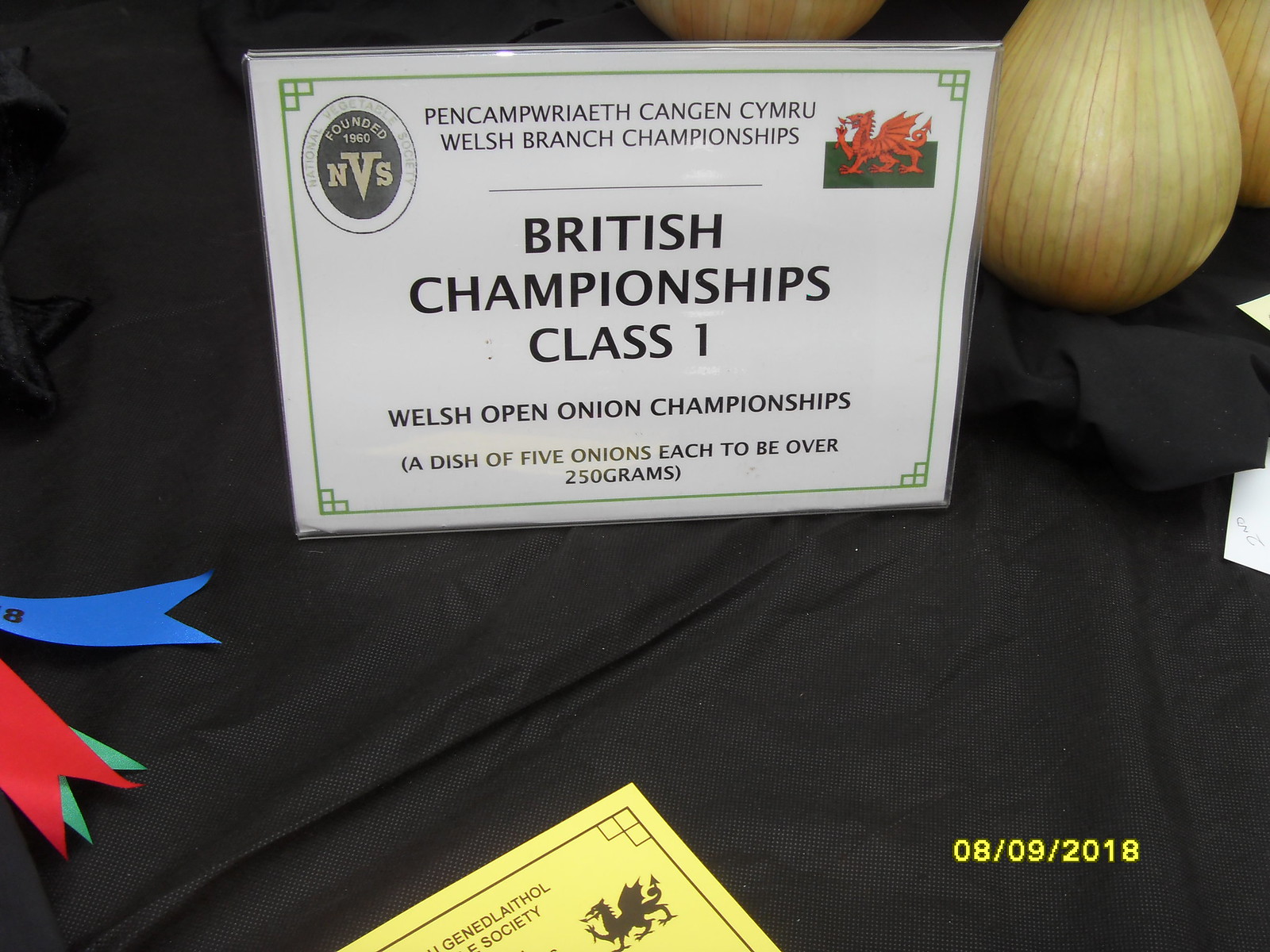The image is a detailed, close-up photograph of a tabletop exhibit at a competition. The table is draped with a wrinkled black cloth, providing a backdrop for the items on display. Prominently featured is a white card in a plastic holder, propped up vertically. This card, oriented horizontally, contains several pieces of text: "British Championships Class 1" and beneath it in smaller letters, "Welsh Open Onion Championships." A yellow date at the bottom reads "08/09/2018."

In the right corner of the background, there are three large yellow onions, part of the display. To the left, we see the ends of blue, red, and green ribbons. Another piece of paper with a black dragon emblem, likely indicating affiliation with the National Vegetable Society (NVS), is visible at the bottom of the frame. The text reveals that NVS was founded in 1960 and the competition, titled "Pen Campreith Cymru Welsh Branch Championships," requires a dish of five onions, each weighing over 250 grams.